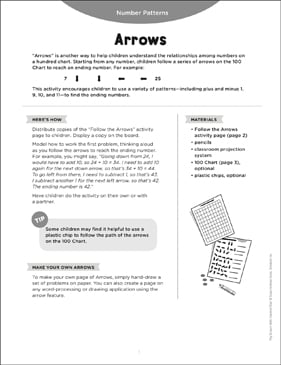The image appears to be a page taken from a child's math workbook or instructional manual, presented entirely in black and white. At the top of the page, there is a grey semi-circle within which the title "Number Patterns" is displayed in white font, followed by the heading "Arrows" in black text beneath it. The blurred text below these headings is largely illegible, but part of it includes an explanatory paragraph that introduces the concept of arrows in the context of number patterns. A notable tip suggests that children may find it helpful to use a plastic chip to follow the path of the arrows on a hundred chart.

The layout of the page includes two main columns of text that are too small to be read clearly. On the right side, there is a bulleted list, possibly labeled "Materials," although specific details cannot be discerned. Additionally, a shaded bubble containing another tip is visible on the left side of the page. The visual components comprise a diagram featuring two sheets of paper laid out with grid patterns, a series of arrows, and a pencil. A partially filled-out questionnaire or example problems can be seen among these drawings. There is also some writing along the right-hand margin, likely indicating publisher information. 

Overall, the page combines textual instructions with visual aids to teach children about number patterns and arrows, suggesting the use of hands-on materials like plastic chips to enhance understanding.